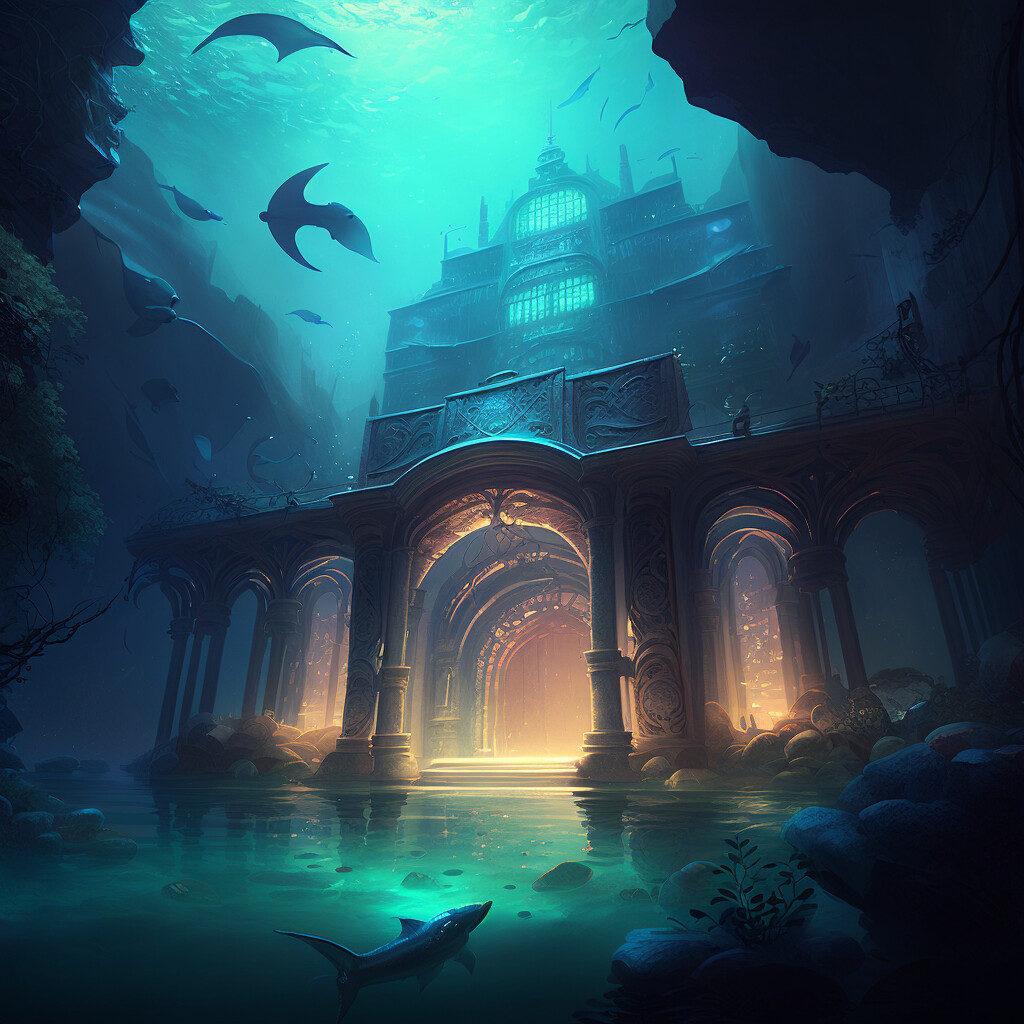This detailed, computer-generated image depicts an enchanting underwater scene, potentially from a digital animation or a painting. Prominently in the foreground, a glowing greenish water area reveals a dolphin-like creature swimming gracefully. The scene is set at night with a dark blue sky and is dominated by a magnificent, multi-storied castle or palace, complete with steps leading into the water. The castle, approximately four or five stories high, features an entrance resembling a Norman window and is adorned with columns, archways, and a steeple at the top. The lower floor of the castle emits a golden reflection from its columns, casting an eerie glow throughout the structure. Surrounding the castle are rocks, boulders, and plants, adding to the naturalistic underwater environment. Small fish and other creatures swim near the top of the image, where light filters in through the water, creating a lighter blue hue. This meticulously crafted illustration beautifully merges architectural elegance with marine life, evoking a magical underwater world.